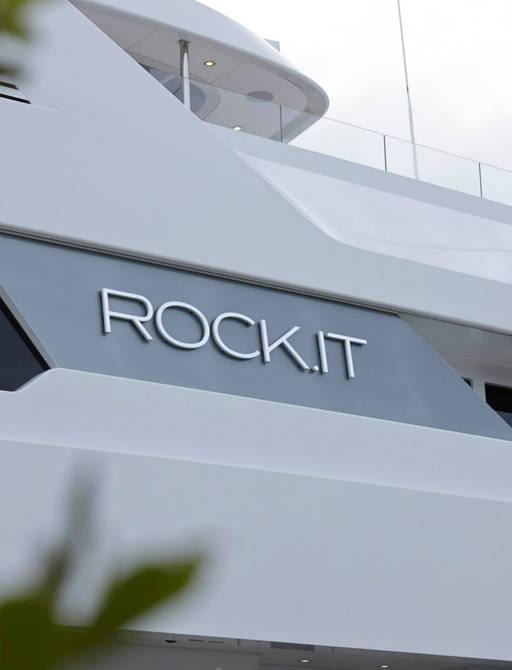This image is a detailed close-up of a portion of a large yacht named ROCK.IT. The yacht's name, affixed to the side in bold, white 3D letters, stands out prominently against a slate gray background shaped like a slanted rhombus. The yacht itself is primarily off-white, featuring sleek, indented curves that contribute to its modern and sophisticated appearance. From this angle, you can see that the yacht has at least three stories. The top story includes a glass-walled balcony with a white canopy supported by metal rods. Some of the lights on the yacht are turned on, indicating interior activity. Additionally, a long white pole extends upwards in the background. The base of the image has a blurry hint of greenery, possibly a bush or small tree. The photo was taken during the daytime, providing clear visibility of the yacht's elegant and detailed design.